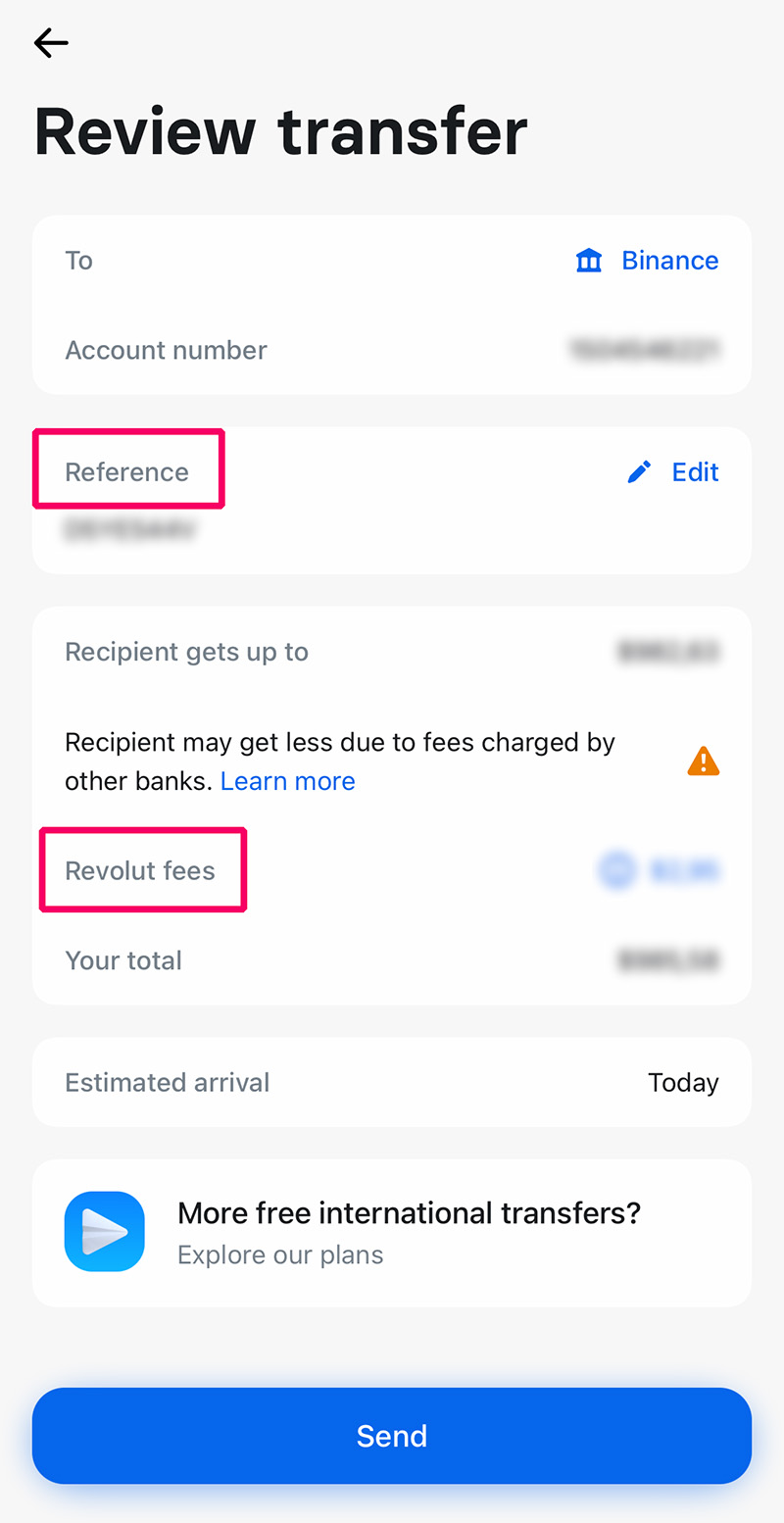A detailed screenshot of a mobile banking app interface, likely from a financial transfer review screen, is depicted. At the very top, there is a left-facing black arrow, indicating a back navigation option. Directly beneath it, the header "Review Transfer" is prominently displayed in black text.

The main body of the interface is segmented into several rectangular sections with rounded corners. The first section begins with the text "To" at the top, adjacent to a light blue bank icon on the right, which is labeled "Binance." Below this, "Account Number" is mentioned in dark gray or light black text, though the actual account number is blurred out for privacy.

The next rounded rectangular box reads "Reference," highlighted in a pinkish-red square. To its right, there is an editable option indicated by a blue pencil icon and the word "Edit." Just beneath this section, additional information is present but blurred out.

Continuing down, the next section is labeled "Recipient Gets Up To," with the corresponding amount on the right side also obscured. Following this, a note in smaller text warns, "Recipient May Get Less Due To Fees Charged By Other Banks," with a clickable "Learn More" link in blue text.

Below this advisory, an orange-filled rectangle with a white exclamation point signals important information. Accompanying this, the text "Revolt Fees" is encased in a pinkish-red rectangle. This is followed by another blue text block, which is also blurred. Adjacent to these sections, "Your Total" is listed, with the specific amount again blurred on the right side.

Near the bottom of the screen, another rectangular box states "Estimated Arrival Today," indicating the expected arrival time of the transfer. The section underneath features a blue rounded-cornered square icon with a white paper airplane, signifying forwarding action, next to the text, "More Free International Transfers. Explore Our Plans."

Finally, at the very bottom of the interface, a solid blue bar with white text stands out, displaying the "Send" button for completing the transfer.